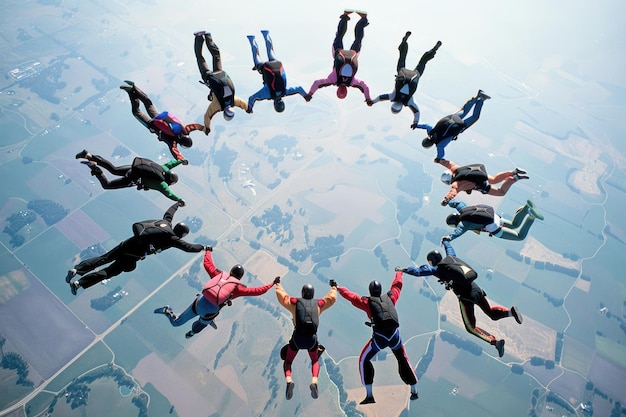The vibrant photograph captures a thrilling overhead view of a group of skydivers in mid-air, forming a tight, hand-held circle. Suspended in the sky, their colorful jumpsuits—including shades of red, blue, green, purple, beige, and orange—contrast strikingly with their uniform black helmets and parachute packs. The image, shot in landscape orientation, offers a breathtaking glimpse of the rural landscape below, with scattered roads, houses, farms, and swathes of trees, all veiled under a light fog. Comprising approximately 12 to 14 individuals, the skydivers' formation resembles a clock face, symbolizing a moment frozen in time before they eventually release their parachutes and drift apart. The scene exudes excitement and unity, capturing the shared thrill of their descent from the plane above.